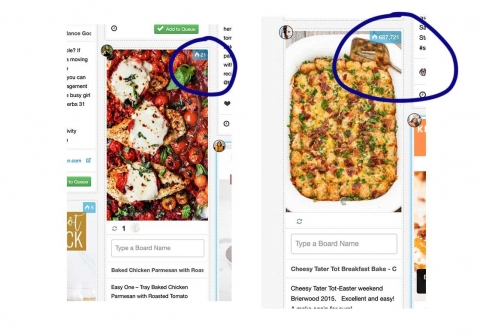The image showcases two distinct meals in a compact format. The first meal, displayed vertically on the left, appears to be baked chicken parmesan surrounded by roasted tomatoes and topped with melted cheese. The incomplete text beneath the dish suggests it is a simple and appetizing option. Above this image, a small symbol of a house marked with the number 21 can be seen in the upper right-hand corner. Both sides of the image contain cut-off information.

The second meal, positioned next to the chicken parmesan on the right, highlights a cheesy tater tot breakfast bake that looks incredibly inviting. This dish is potato-based with visible text praising its ease and excellent taste, labeled "cheesy tater tot, easier weekend."

At the top of the image, there's a green box with a check mark, though its purpose remains unclear. The information accompanying the second image is cut off, making the details obscure. Despite the confined space and truncated text, the photographs emphasize the delicious appeal of both meals.